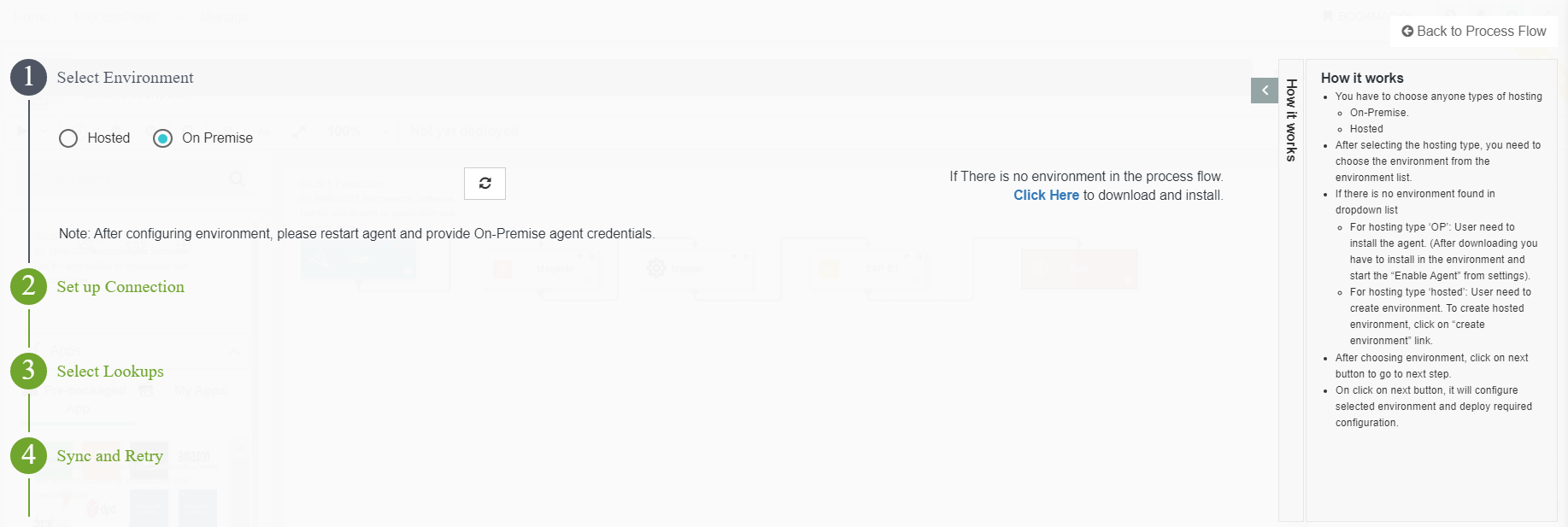Here's a cleaned up and detailed caption for the described image:

---
Screenshot of a website interface depicting the initial phase of a four-step setup process. The user is currently on Step 1, which is to select an environment—either hosted or on-premise. The interface provides options for the user to choose their desired hosting type. Sequentially, Step 2 involves setting up the connection, Step 3 focuses on selecting lookups, and Step 4 covers synchronization and retry procedures.

On the right side of the interface, there is a prompt stating, "If there is no environment in the process flow, click here to download and install." Additionally, a sidebar labeled "How It Works" offers a detailed bullet-point guide clarifying the process. It instructs users to select either on-premise or hosted as their hosting type. 

For on-premise:
1. Choose the environment from the provided list. 
2. If no appropriate environment is found, download and install the necessary agent.
3. Install the environment and enable the agent from the settings.

For hosted:
1. Create a new environment by clicking the "Create Environment" link.
2. Once the environment is selected, proceed by clicking the "Next" button.

Upon clicking "Next," the system will configure the selected environment and deploy the required configurations.

---

This caption provides a comprehensive and clear description of the interface and the step-by-step process depicted in the screenshot.